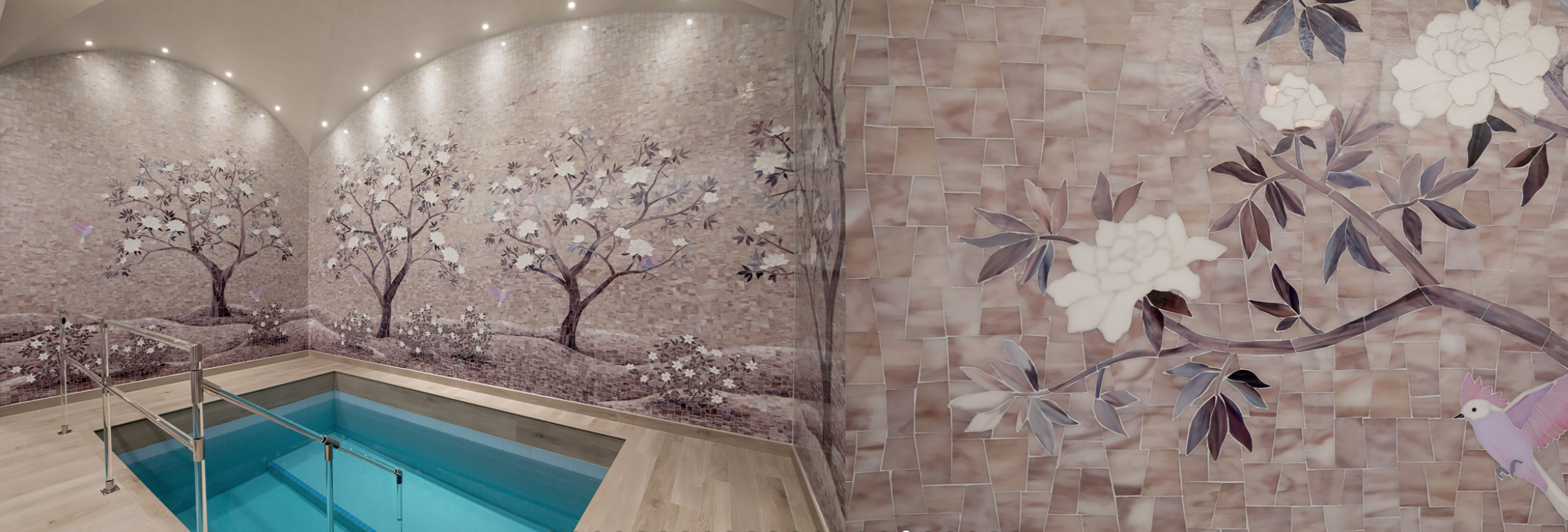This indoor relaxation area, captured in a rectangular colored photograph, appears to be part of a serene spa environment. The room is square-shaped and features elegant lavender walls adorned with small, evenly spaced white lights that create a tranquil ambiance. These lights are positioned above the walls in gentle arcs, enhancing the room's serene atmosphere. The walls themselves have a brick-like texture, and they are decorated with images of delicate Japanese-style trees that bear large, white flowers and some green leaves, set against a backdrop of rolling hills.

The floor of the room is made of a light wooden surface that surrounds the main focal point: a small, in-ground pool. This pool, though resembling a swimming pool in its built-in design, is more akin to an oversized hot tub or therapy pool in size. A metal handrail on the side of the pool provides support for those entering the water, which seems to be approximately eight feet deep. The overall ambiance of the room exudes tranquility and is designed for relaxation and therapeutic purposes.